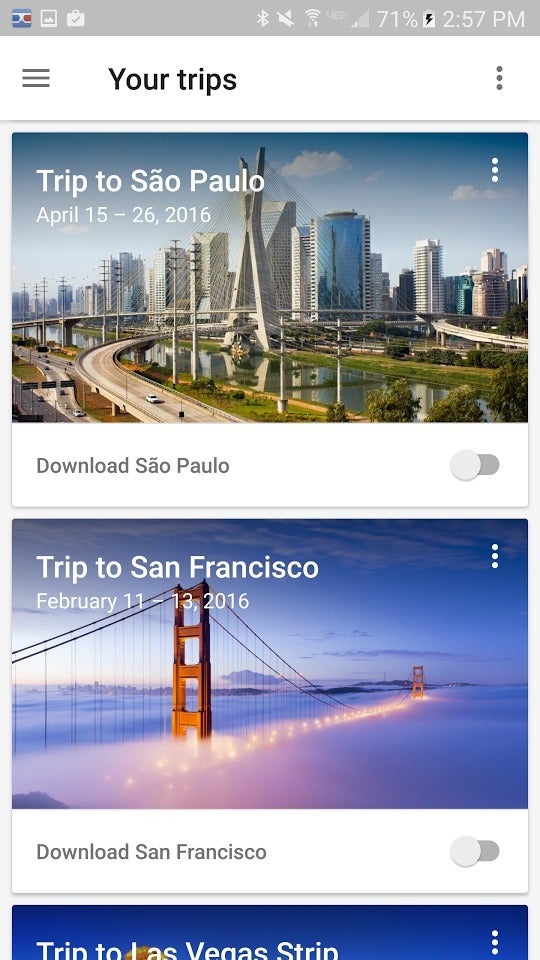The top left corner of the image displays a blue icon resembling a pair of glasses, alongside various status symbols such as a gray bar, Bluetooth, speaker, Wi-Fi or 4G, and a battery indicating a 71% charge with a lightning bolt. The timestamp reads "7:00 PM."

The left section of the image features a trip to Sao Paulo, with visuals depicting Sao Paulo’s skyscrapers, bridge, railway, and river. The travel dates are April 15 to 26, 2016, accompanied by a "Download Sao Paulo" button and a checkmark confirming the trip.

On the right, there's information about a trip to San Francisco, featuring an image of the fog-covered Golden Gate Bridge. The travel dates for San Francisco are February 11 to 13, 2016, alongside a "Download San Francisco" button.

Additionally, there is a segment mentioning a trip to Las Vegas, set against a blue background. Overall, the image appears to be a section of a travel website showcasing different travel destinations and their details.